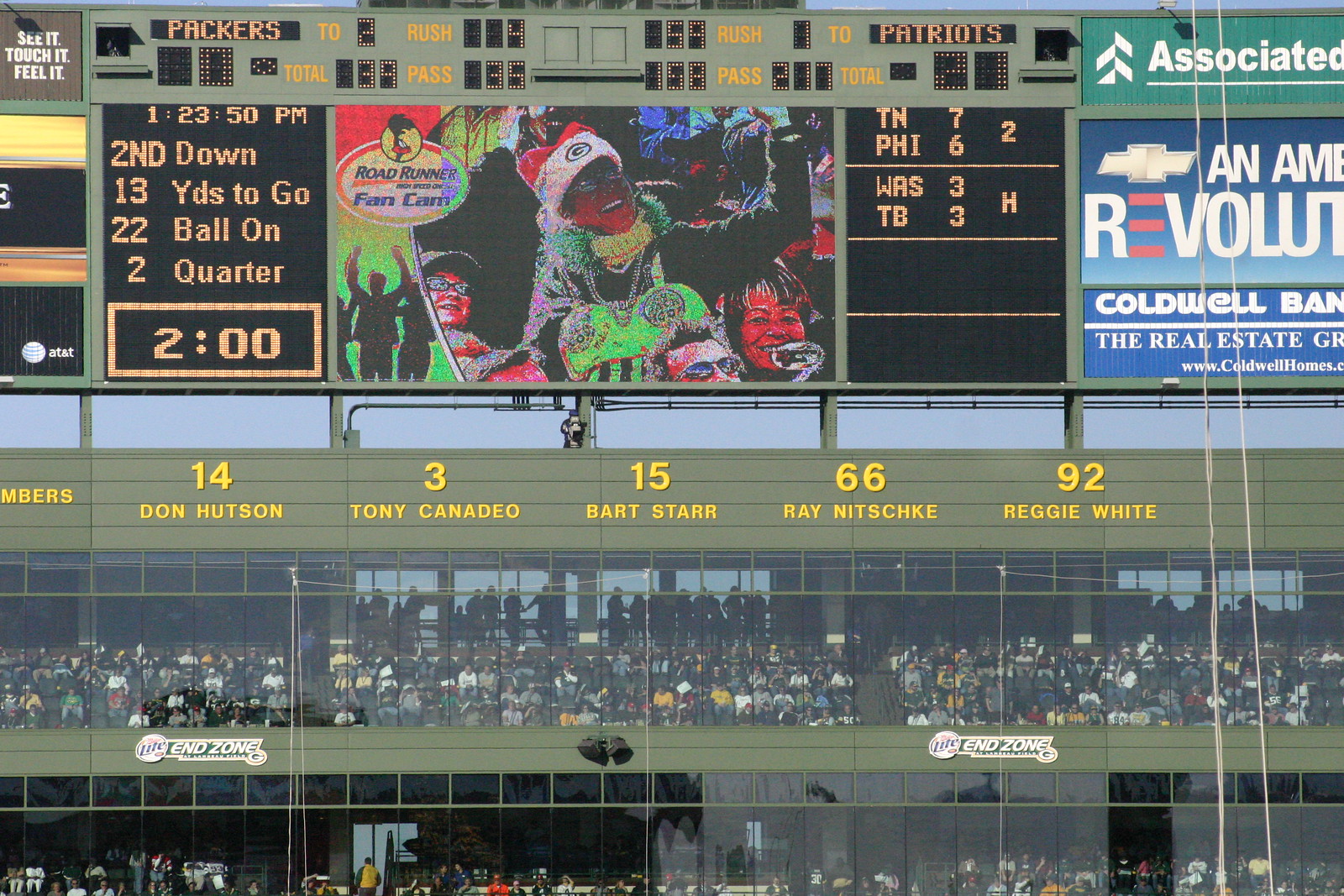The image captures the electrifying atmosphere of an NFL game between the Green Bay Packers and the New England Patriots, as seen from within the stadium. The focal point of the photo is the Jumbotron, prominently displaying a fan decked out in festive Christmas attire, including red and green clothing and a Santa hat. Surrounding him are detailed game stats: the Packers have the ball on second down with 13 yards to go and 22 yards to the goal line, while the Patriots' game stats are also displayed. The scoreboard features ads, including a Chevrolet logo and signs for American Revolution, Green Associated, and Codwell Bank Real Estate.

Above the stats, in vivid yellow letters, are the names of Packers legends: 14 Don Hutson, 3 Tony Canadeo, 15 Bart Starr, 66 Ray Nitschke, and 92 Reggie White. The image also captures the stadium's green-themed seating, packed with fans. The stands appear to be divided into two rows, with glass separating sections, adding to the vibrant, enclosed feel of the venue. The silhouetted crowd collectively enhances the game's lively atmosphere, making it clear this is a high-energy NFL event.